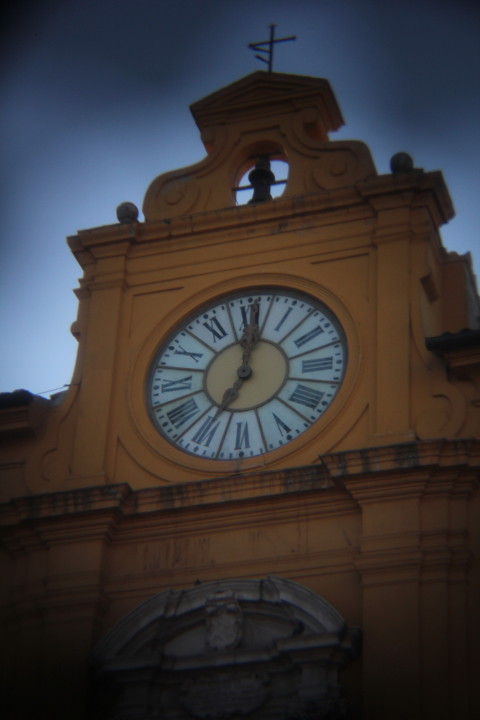This image features a tall, ornate church bell tower with a cross perched at the very top, silhouetted against a sky that suggests an impending storm or a setting sun, possibly indicating it is evening. Dominating the center of the structure is a large, analog clock exhibiting black Roman numerals on a white face, encircled by minute dashes and displaying the time as seven o’clock. The clock's hands are robust and brown, while the clock’s center is marked by a striking yellow. Above the clock sits a large bell in a recessed cubby. The tower itself, constructed in a golden brown or honey mustard hue, displays intricate woodwork with curled designs and small knobs along its edges. The exterior paint is faded, revealing black streaks that may be dirt, especially notable on the ledges below the clock. The structure culminates in a detailed stone foundation at its base.